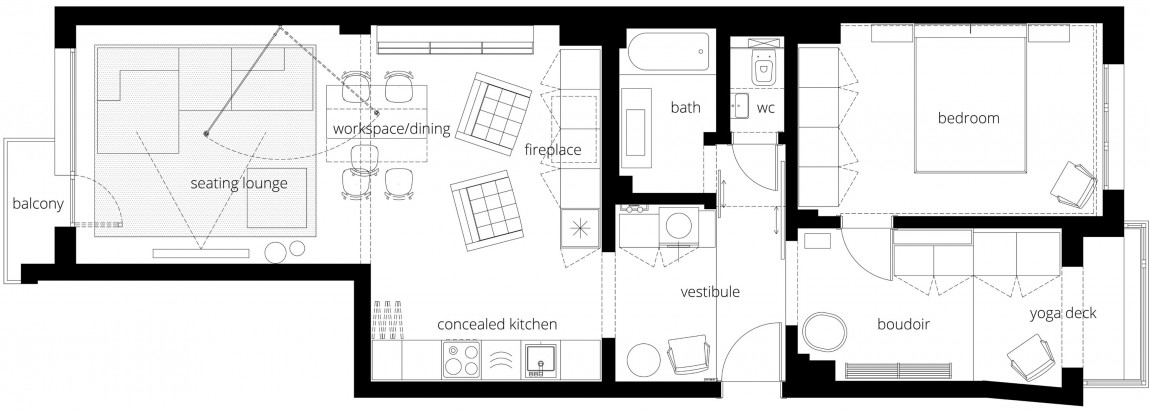The architectural room layout presents a horizontally oriented building. The main section of the building spans wider than the left-hand portion, which forms a large notch out of the larger back area. At the rear of the building, there is a door and window imagery, leading to a marked balcony outside the room.

To the right, the layout features a seating lounge depicted by lines representing seating areas, along with a wall-mounted TV. Adjacent to this seating lounge is a workspace and dining area, illustrated with the outline of a table and chairs. Further right, there are two overstuffed chairs positioned in front of a fireplace.

The bottom edge of this room encompasses a concealed kitchen equipped with a range and sink. Notably, there is no dividing wall between the seating lounge and the kitchen. To the right of the kitchen, an entryway leads to a vestibule where the front door is shown at the bottom of the image. The vestibule includes a round table next to a cushioned chair, and above the chair, an outline suggesting a washer and dryer.

Behind the vestibule is a bathroom, which connects to a small water closet or toilet area via a wall. Two rooms positioned to the right of the bathroom and bath area include a bedroom with a large bed, closet, and a chair. This bedroom provides access through a door to a boudoir, and adjacent to this room is a yoga deck leading to another balcony.